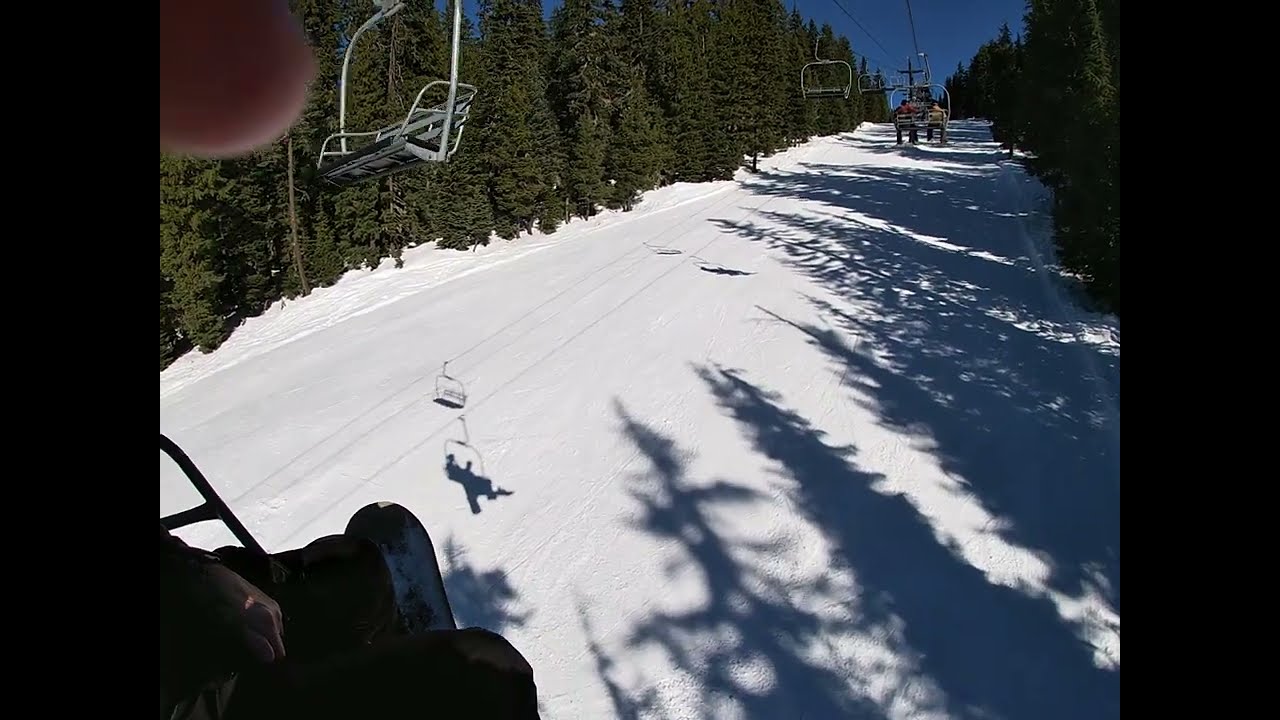This full-color photograph, taken from a ski lift on a bright, sunny winter's day, captures a picturesque snowy scene at a ski slope. The image is horizontally rectangular with thick black borders on the left and right sides. Tall pine trees flank the image, creating a natural frame, while their long shadows stretch across the pristine white snow beneath.

The photographer is aboard the ski lift, evident from their finger partially obscuring the lens in the upper left corner and their shadow in the snow below. In the center of the image, the ski lift cables extend into the distance, with empty lifts moving in the opposite direction. A lift farther ahead carries two people, blurred slightly by the distance. The photographer's other hand rests in their lap, casting a shadow that is also visible on the snow. The scene showcases a clear blue sky and the dense greenery of the pine trees, contrasting with the white expanse of snow, epitomizing a crisp winter day on the slopes.